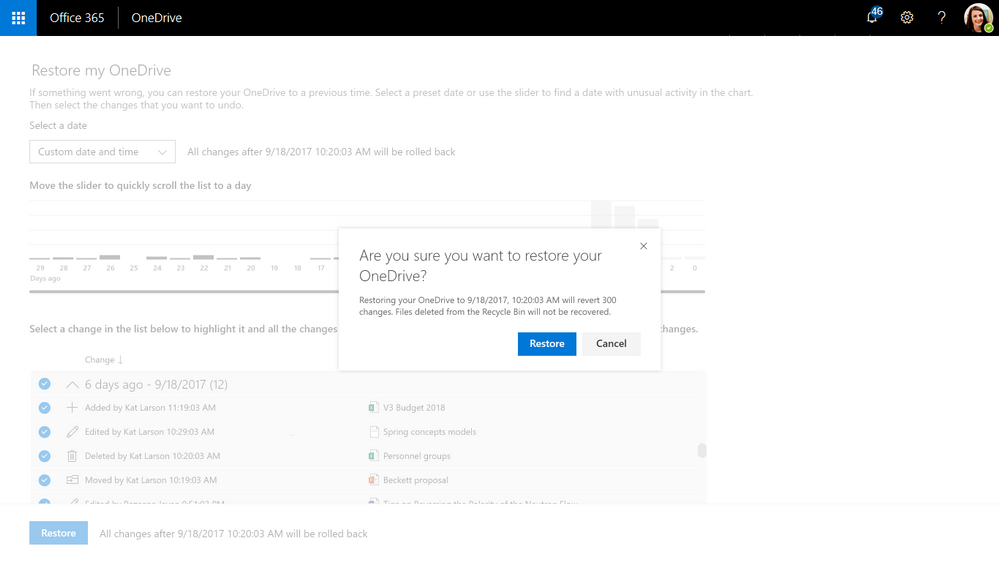In the image, there's a screenshot of an Office 365 OneDrive interface. At the top left, there are nine square dots arranged in a grid, indicating a menu. The top banner is black with the text "Office 365 OneDrive" displayed in white font. To the right, there is a notification icon with a count of 46 notifications. Adjacent to it, there's a gear icon representing the settings menu, and a display image of a woman, likely the user’s profile picture.

Beneath the banner, the main content shows a faint pop-up window titled "Restore my OneDrive." This window allows users to revert their OneDrive to a previous state if something has gone wrong. The interface displays options to reset by selecting a date, with the example showing a date of September 18, 2017. There's a warning message that reads, "Are you sure you want to restore your OneDrive? Restoring your OneDrive to 9-18-2017 at 10:20:03 AM will revert 3,300 changes. Deleted files from Recycle Bin will not be removed." 

At the bottom of the pop-up, there are two buttons: a blue "Restore" button and a gray "Cancel" button. The background of the website under the pop-up is indistinct but suggests a typical file listing, indicating the context of where changes will occur.